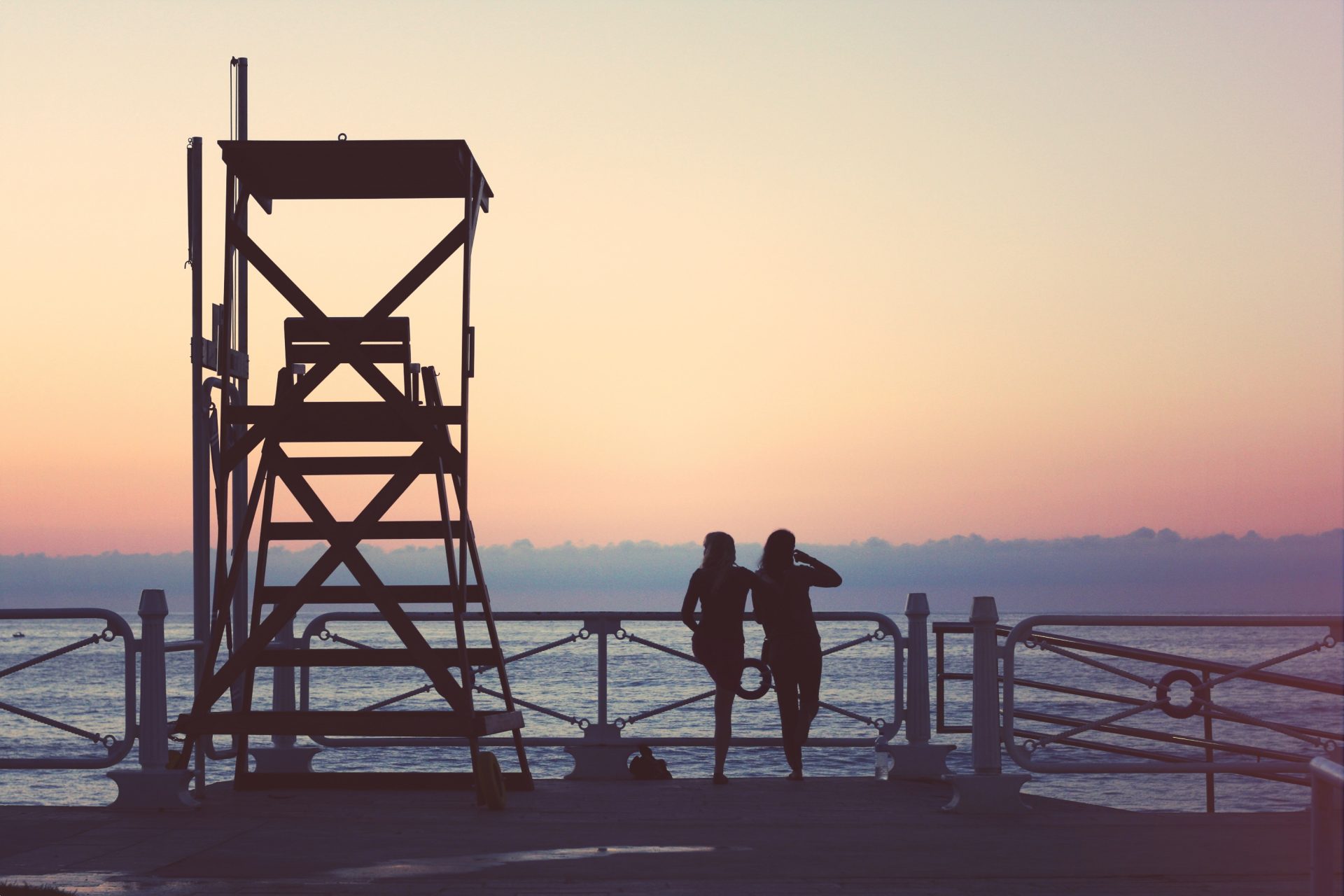In the photograph, there is a scenic view of a harbor or beach during sunset, captured in landscape mode. The sky takes up approximately 60% of the image, exhibiting a beautiful gradient from a pale, light color at the top, transitioning through shades of yellow, and culminating in a deep reddish-orange hue near the horizon. Silhouetted against this vivid sky are the dark outlines of trees.

Situated near the left side of the image, a lifeguard tower stands tall, constructed from either metal or wood, with a stairway leading up to it. It features a place to sit, and its structure is bathed in the glowing, gradient light of the sunset, rendering it almost entirely black like a silhouette.

In the center of the scene, two women with long hair can be seen standing by a steel fence, which extends from the left below the center to the right edge of the photograph, marking the water's perimeter. They appear to be on a boardwalk or pier, engrossed in the view of the ocean before them. The light and angle create compelling silhouettes of the women, one of whom has her hand near her face, and both of them gazing in different directions, lost in contemplation against the backdrop of the serene, blue waves of the ocean beneath the enchanting twilight sky.